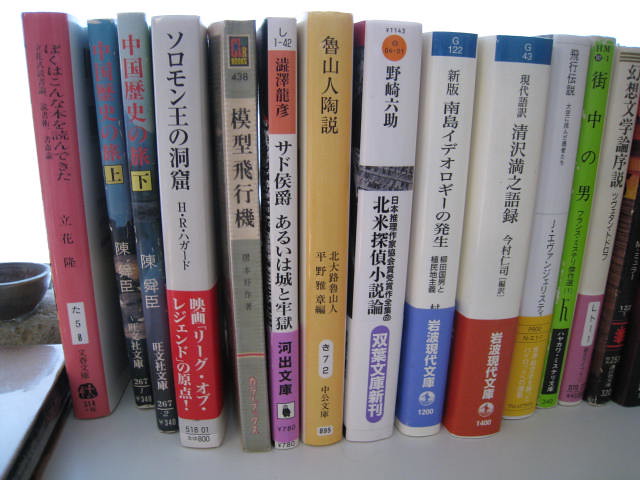This photograph features approximately 15 books standing upright on a white countertop, possibly resembling a shelf or table. The books, primarily paperbacks, display spines with what appears to be Chinese or Japanese characters, indicating they are written in an Asian language. To the left of the books, there's a partial view of a brownish-gray porcelain bowl and what might be a square, shiny silver plate or a laptop.

The books vary in colors and sizes but maintain a similar height, suggesting they could be around 6 inches tall. Starting from the left, the spines are predominantly red, followed by two books featuring blue cityscape images. The collection continues with a white book with a red band, a gray book, and a white spine with orange and pink stripes. There are also yellow, green, and several white spines separated by thin bands of colors like red, blue, and yellow. Some books share similarities in design, hinting they might belong to a series. The white background and bright lighting, possibly from a window, highlight the colorful arrangement and the detailed calligraphy on the spines.